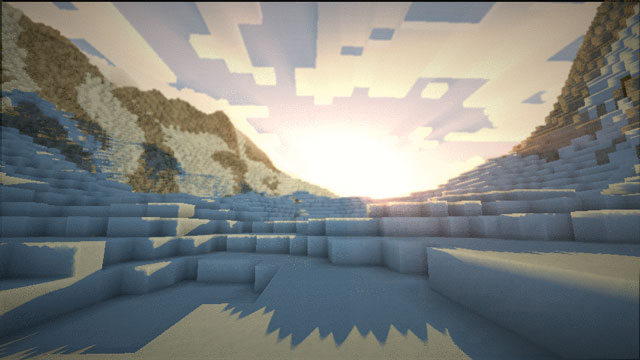This image appears to be a screenshot from Minecraft, showcasing a detailed and immersive landscape. The scene is set in a vast valley nestled between mountains that flank both the left and right sides. The perspective is taken from within the valley, providing an upward view of the blocky mountains. The mountains display an earthy brown hue near their summits, contrasted by patches of white on their sides, possibly indicative of snow or light-colored rock. 

The valley floor is covered in a whitish terrain, enveloped by shadows cast by the surrounding peaks. In the background, the sky is dotted with blocky, white clouds drifting towards a focal point where a luminous light source, presumably the sun, is located. This bright light suggests the time of day is either sunrise or sunset, casting an ethereal glow over the entire landscape and creating dynamic shadows across the scene. The image captures the quintessential blockiness of Minecraft, highlighting both the simplicity and beauty inherent in its design.